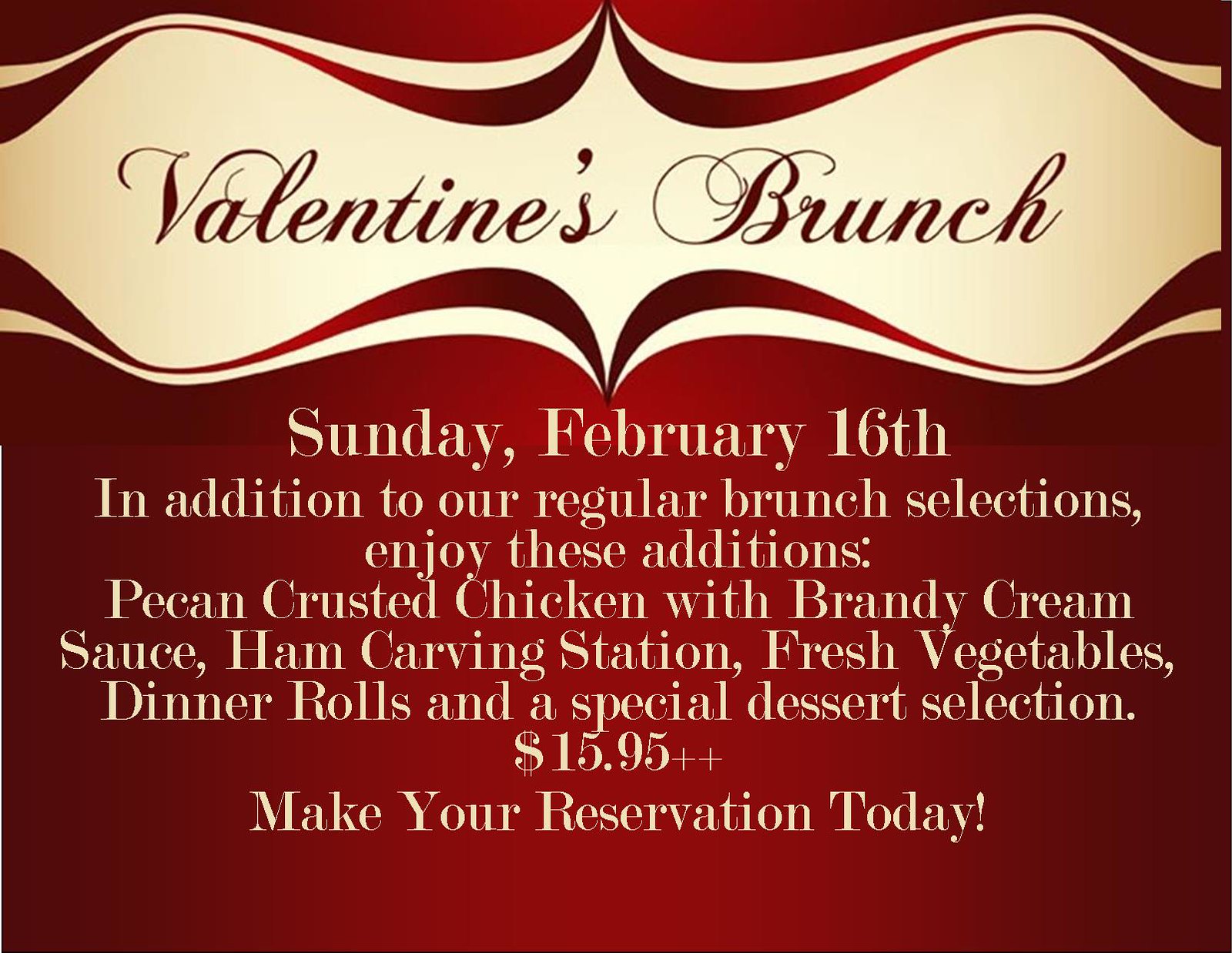This promotional flyer is designed for a Valentine's brunch set against a rich red background. The top third features a sophisticated tan swirl design, which overlays a beige strip bordered with red curvy lines, adding an elegant touch. In deep burgundy cursive, it announces "Valentine's Brunch," followed by the date, Sunday, February 16th, printed in a complementing script. Below this, the flyer details the brunch offerings: in addition to the regular selections, there will be pecan-crusted chicken with brandy cream sauce, a ham carving station, fresh vegetables, dinner rolls, and a special dessert selection. At the bottom, it encourages making reservations, highlighting the price of $15.95++. The entire flyer is cohesive in its use of deep red, beige, and tan colors, creating a festive and inviting feel.